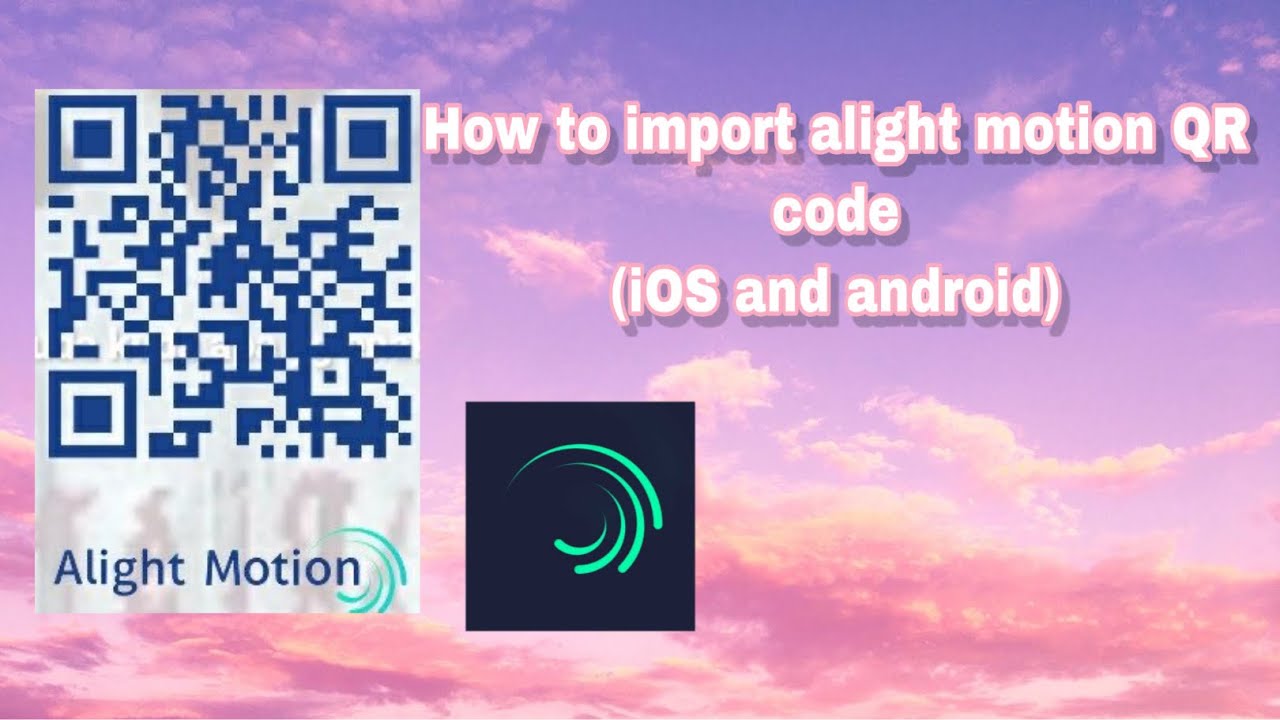The image is an advertisement detailing how to import a Lightmotion QR code for both iOS and Android. The main focal point is a QR code on the left side, accompanied by text that reads, "How to import a Light Motion QR code (iOS and Android)" in white letters with a slight pink border. The text is spread across multiple lines: "How to import a Light Motion QR" on the top, followed by "code" on its own line, and "(iOS and Android)" on the next line. To the right of the QR code, there's a black box featuring the Light Motion logo, which consists of four green swirling lines almost connecting in a circular shape. The background is a surreal blend of a purplish-blue sky transitioning to reddish-orange and pink clouds, creating a dreamy and artificial atmosphere.